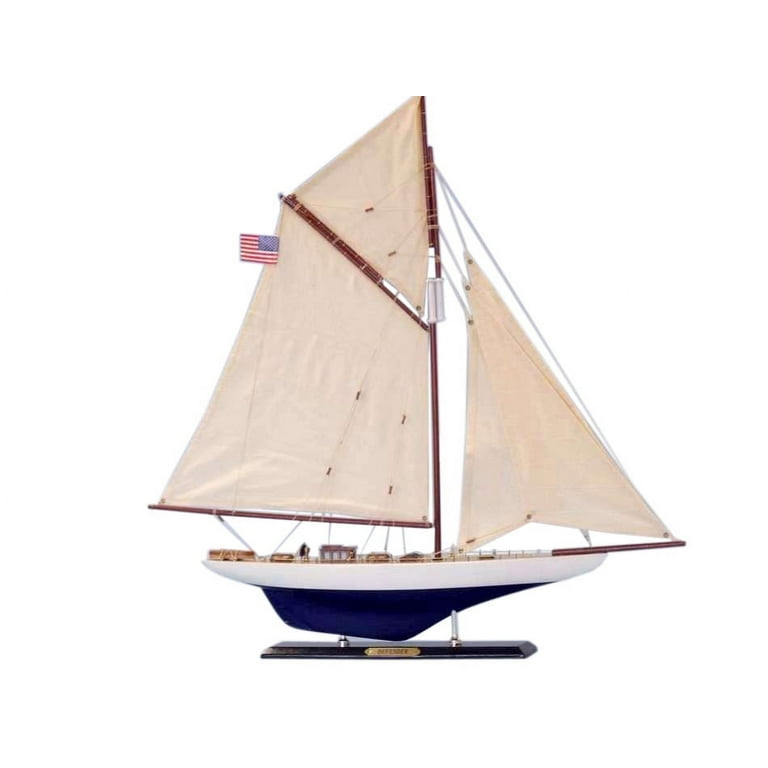This is a detailed photograph of a meticulously crafted scale model sailboat, displayed prominently against a bright white background. The model sailboat, supported by two metal pegs affixed to a sleek black wooden platform, boasts a gold plaque inscribed with indiscernible black lettering. This vessel, viewed from the side, features a blue body with a white upper rim along the waterline. The boat is equipped with three sails—one at the bow and two at the stern—crafted from tan canvas and mounted on dark brown masts. Rigging lines extend from the base to the top of the sails, which are strategically directed by a long brown pole protruding from the front. An American flag proudly flutters from one of the aft sails. The deck includes a small windowed box, seemingly accommodating a staircase to access below deck. Additionally, the vessel's deck is furnished with supplies, enhancing the authenticity of this scale model sailboat.